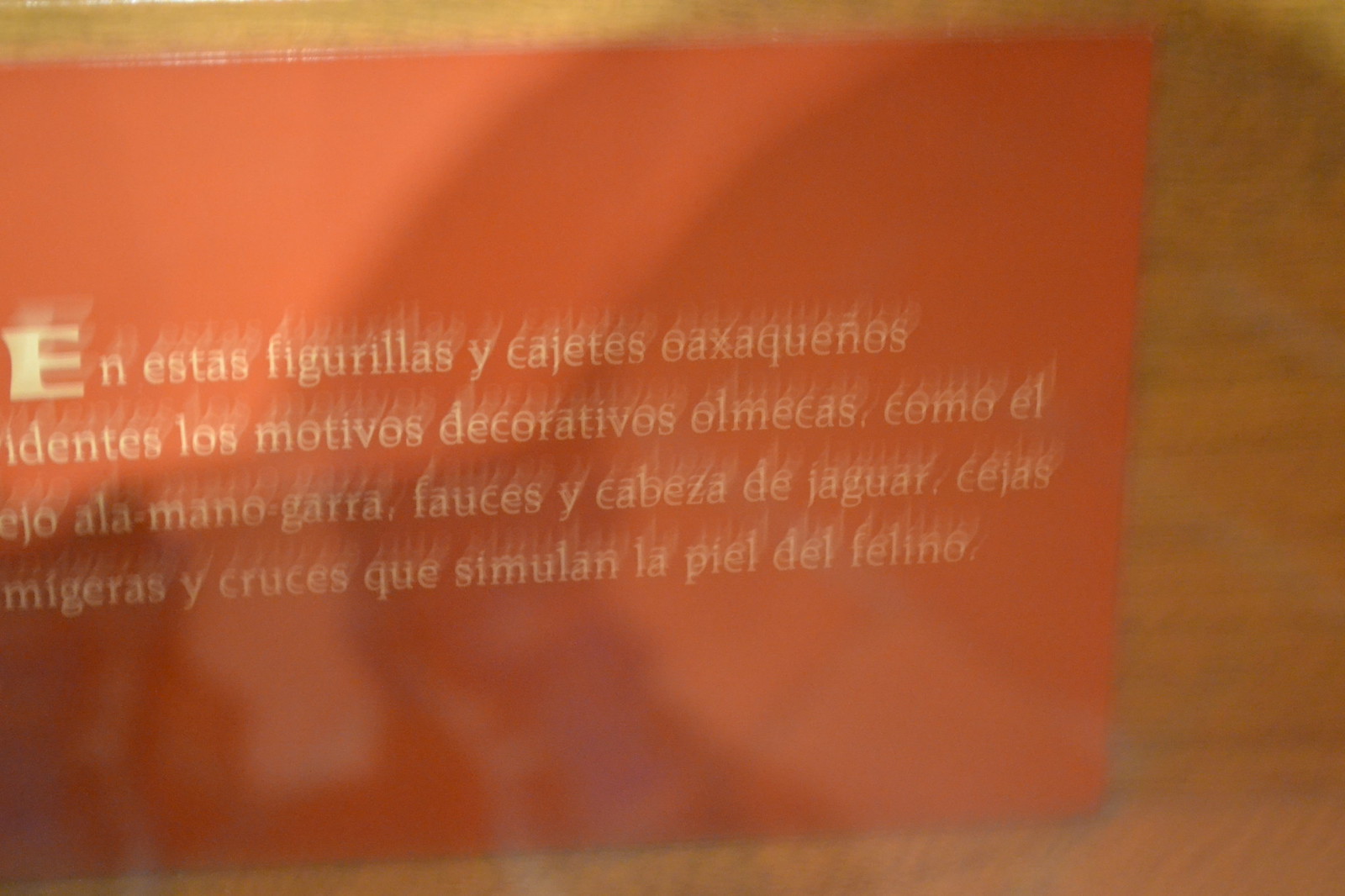The slightly blurred colour photograph depicts a vibrant red banner or card leaning against a light brown brick wall. The banner features text in a creamish off-white color, arranged in four lines, and written in what appears to be a foreign language, possibly Spanish. The text includes the phrase "I en estas figurilas," followed by a large letter "Y" and "Cajetes," with the word "Jaguar" also visible. The banner isn't perfectly horizontal; it tips upwards to the right, revealing a portion of the floor at the bottom right corner of the image. There is a noticeable shadow across the banner, suggesting either the presence of the photographer or another object outside the frame. The text is slightly diagonally ghosted towards the top right, adding to the visual complexity. The overall impression is reminiscent of a sign you might find at an outdoor fair, museum, or gallery, potentially related to animals or a zoo.